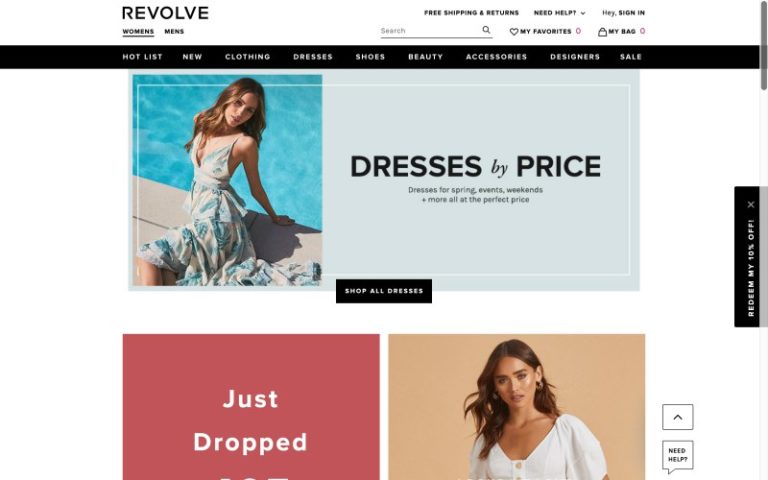Certainly! Here’s a cleaned-up and detailed caption for the image:

---

The webpage from Re-Balt, an online shopping store for both women's and men's fashion, prominently displays its brand name in the upper left corner. Below the logo, there's a navigation bar featuring tabs for 'Women' and 'Men'. Directly beneath these tabs, a sleek black bar provides quick access to various categories: 'Hot List,' 'New Clothing,' 'Dresses,' 'Shoes,' 'Beauty,' 'Accessories,' 'Designers,' and 'Sale.' A visually striking centerpiece image shows a young woman elegantly seated beside a pool, labeled with 'Dresses for...' and a price filter option. Below this main image, another partly visible photo depicts another young woman, suggesting more content further down the page.

---

This caption offers a clear and detailed description of the webpage layout and its visual elements.